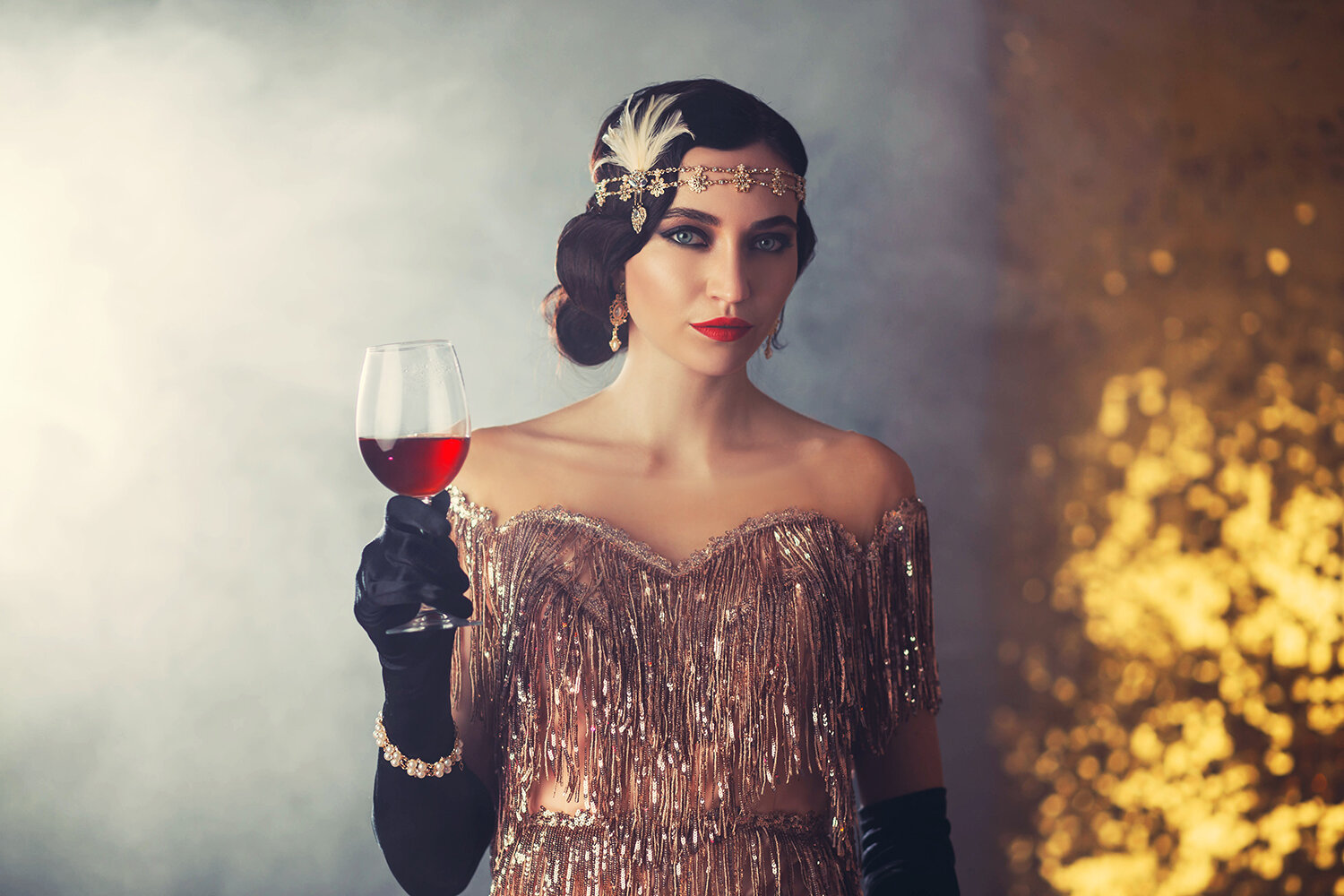In this horizontally rectangular indoor image, likely taken during an extravagant party, the center of focus is a woman dressed in an elegant, flapper-style outfit reminiscent of the 1920s and 1930s. She stands confidently in a room where the background shifts from light gray on the left to a dark gold glittery hue on the right. The details are somewhat blurred, with a hint of a white-colored element in the background and possibly some lit-up decorations resembling gold lights or a lighting display on the right side.

The woman is adorned in a glamorous strapless gown, made of shimmering golden and silver fringe that cascades over a copper-colored fabric. She exudes sophistication with her black hair styled in soft, rolled waves just above her shoulders, and a gold headband decorated with a white feather elegantly rests on the side of her head. 

Her face is artfully made up with smoky eye makeup and deep red lipstick, adding to her vintage allure. She accessorizes with long, elbow-length black gloves and a jewelled bracelet on her right wrist. In her right hand, she holds a clear goblet filled halfway with red wine, heightening the festive and luxurious atmosphere of the scene.